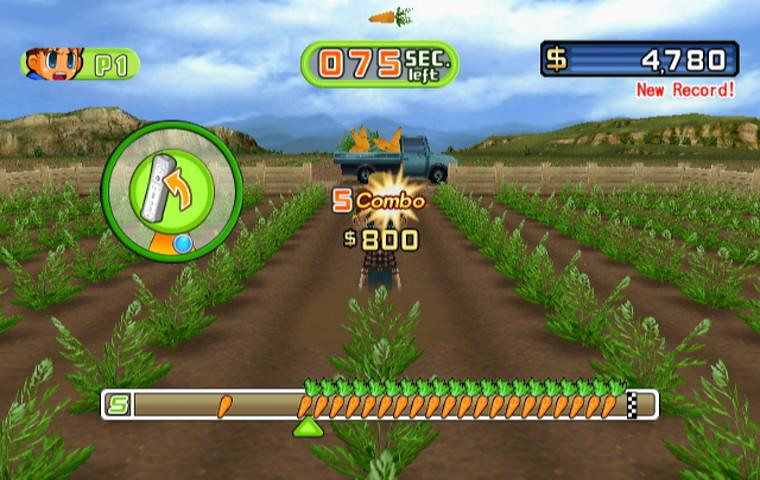The image displays a vibrant, in-game scene from a farming simulation game, likely being played on a computer given the horizontal orientation of the screen. The background features a picturesque landscape with a clear blue sky dotted with fluffy white clouds, and lush green hills and mountains. 

Prominently in the foreground are ten rows of green carrot tops emerging from rich brown soil. The rows are arranged with one central row and two expansive rows stretching back, while the other rows branch out diagonally. Positioned centrally within these rows is a farmer dressed in a plaid shirt and pants. Nearby, there is a flatbed truck loaded with freshly harvested carrots, parked just behind him.

The bottom of the screen features a graphical bar filled with carrot icons. In the center of this bar, it displays "5 combo" and below it, "$800" indicating the player's current achievements. At the top of the screen, it indicates "0.75 seconds left" and displays a large carrot icon above the timer. 

On the left side of the screen is a face icon labeled "P1," suggesting a player identifier. On the right-hand side, a dollar sign is shown with "$4,780" next to it and the phrase "new record" highlighted in red beneath it. 

Mid-left of the screen, there is a round icon with a green circle and an arrow pointing towards a white, TV remote-shaped controller, which possibly functions as a control guide. At the end of the carrot rows, a beige fence marks the boundary of the farm area.